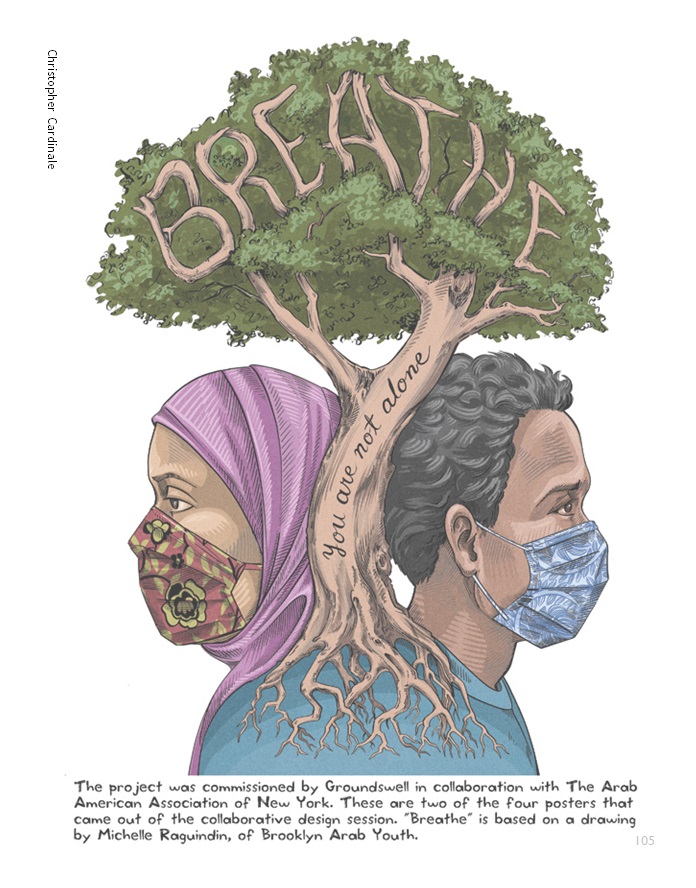The image depicts a vividly painted poster showcasing a large tree trunk growing vertically between two individuals' faces. The tree's leafy green canopy features the word "BREATHE" in light purple letters. Engraved vertically along the trunk in dark letters is the message, "YOU ARE NOT ALONE," with emphasis on the uppercase "U." On the left side of the tree stands a woman with darker skin wearing a purple headscarf and a multicolored green and red face mask. On the right, a dark-haired man with darker skin wears a blue and white mottled mask, with the mask's loop visible over his ear. Both individuals appear to share a conjoined body dressed in a gradient blue top. Their heads are positioned back-to-back, touching the tree trunk, which extends down to its roots, intertwining into their shoulders. At the bottom of the poster, a caption details that the project was commissioned by Groundswell in collaboration with the Arab American Association of New York. This artwork is one of four posters created during a collaborative design session, with "Breathe" based on a drawing by Michelle Ragudin of Brooklyn Arab Youth. Additionally, the name "Christopher Cardinal" appears in the upper left-hand corner, further attributing the piece.